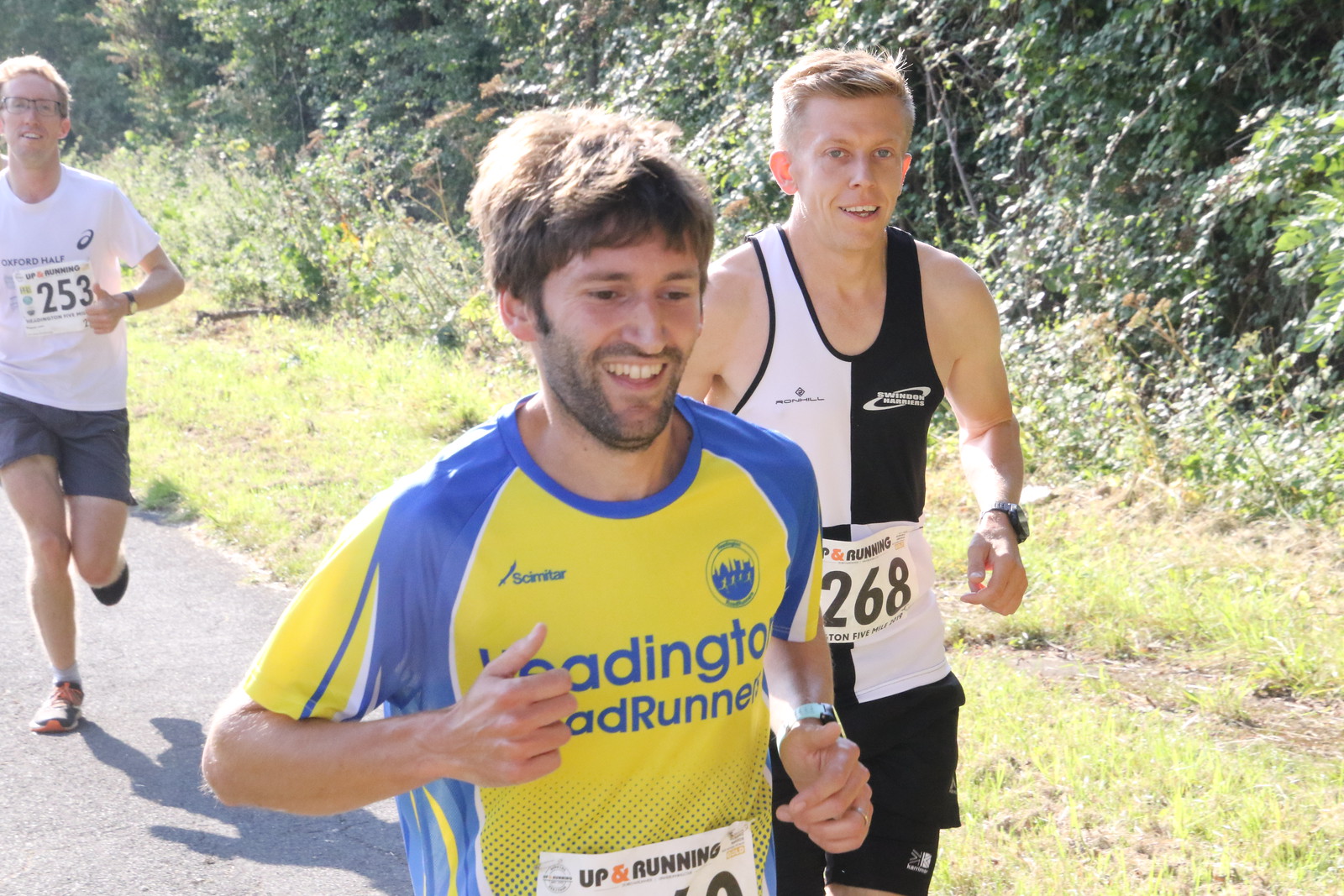This photograph captures a vibrant outdoor scene of three men running on a sunlit road, likely participating in a race or marathon. The runner in the foreground is wearing a yellow shirt with blue accents and has brown hair, although his race number is not visible. Close behind him is a smiling man clad in a black and white outfit, bearing the number 268. The third runner, slightly further back, is dressed in a white shirt and gray pants, wearing glasses, and features the number 253 on his chest. Each runner appears upbeat and focused, contributing to the lively atmosphere of the competition. The road beneath them appears to be asphalt, marked by the sunlight casting shadows. To the right of the road, the landscape is lush and verdant, with green grass extending into a backdrop of trees, plants, and leaves, all illuminated by the bright sunlight.